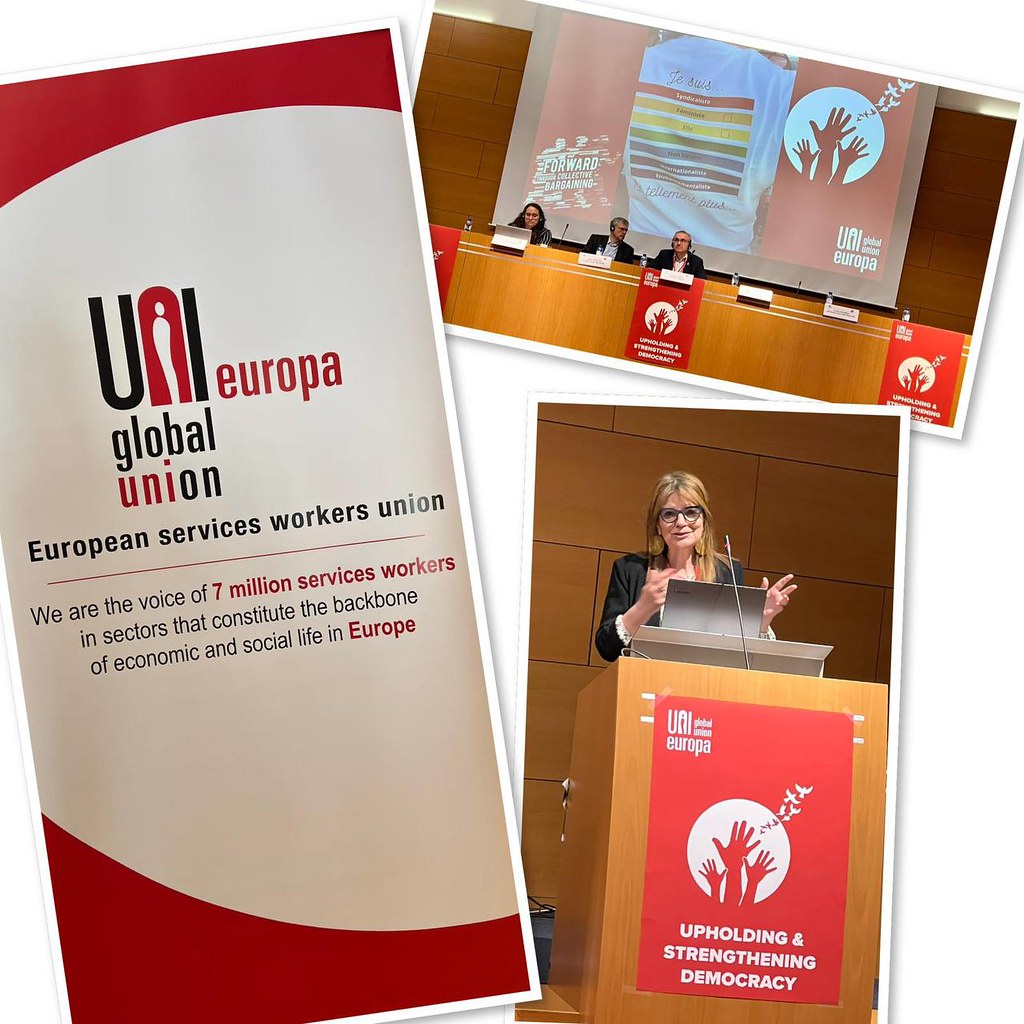The image is a detailed collage centered around a conference organized by Uni Europa, Global Union. On the right side, a woman stands at a podium with her laptop, addressing the audience. The podium prominently displays a red poster with white text that reads "UUI Europa, Global Union" and "Upholding and Strengthening Democracy." Below the podium, there is more text on the left side that says "European Services Workers Union" and "We are the voice of 7 million service workers in sectors that constitute the backbone of economic and social life in Europe." To the right, a landscape photograph captures a panel of three speakers seated at a long booth with a projector screen behind them. The left side features an infographic or poster with the same Uni Europa, Global Union branding and a distinct red icon integrated into the letter 'N,' symbolizing the union. The overarching theme of the collage emphasizes the union's focus on supporting service workers and promoting democracy within Europe's economic and social framework.